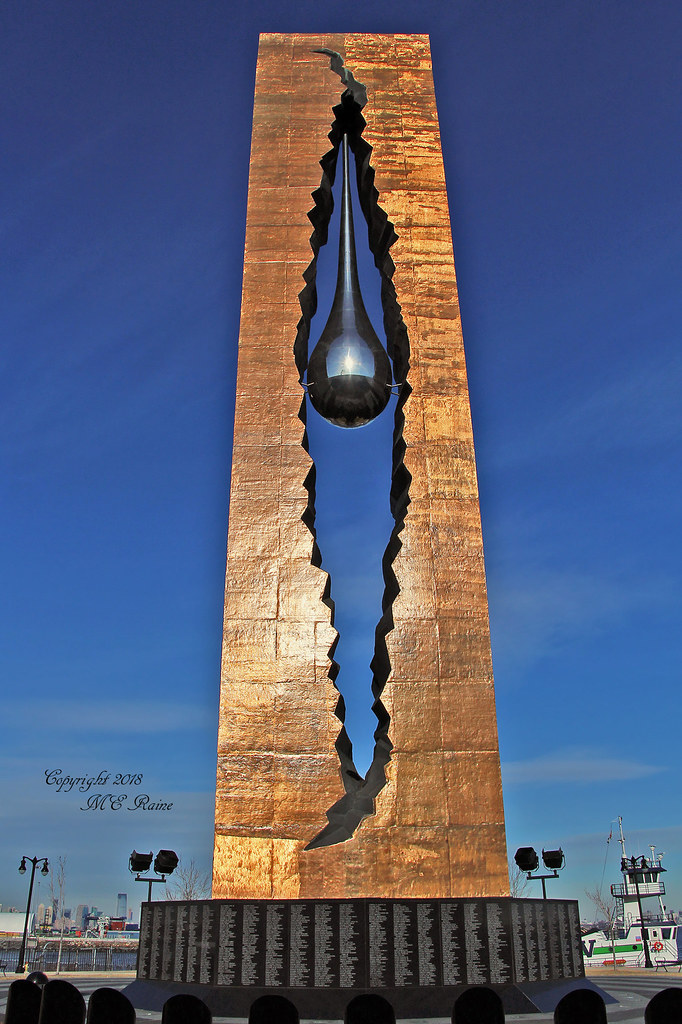The image captures the Teardrop Memorial Monument, a tall, vertically aligned rectangular structure made of shiny granite-like stone, standing prominently on a black circular base. The monument, painted in shades of bronze or gold, features a dramatic central crack that splits the structure, revealing a teardrop-shaped object, likely made of glass or metal, suspended from the top. The setting includes a clear blue sky with subtle white clouds, suggesting a serene and open environment. In the background, city buildings, boats, and lights—streetlights or stage lights—hint at a waterfront location. The bottom of the monument's base curves gracefully, displaying inscribed names or words. The image also has overlaid text on the bottom left corner, reading "Copyright 2018, M.E. Rain." The dominant colors in the picture are gray, blue, silver, various shades of gold, bronze, brown, black, and white, contributing to the overall detailed and striking appearance of the monument.